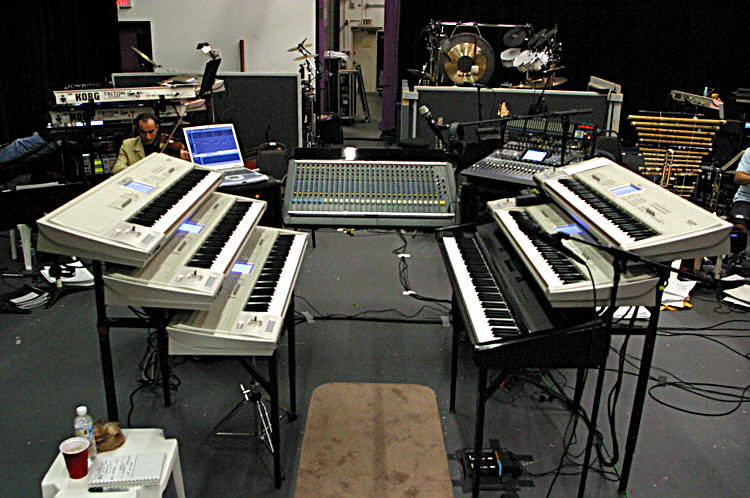The image depicts a well-equipped recording studio, featuring a variety of musical instruments and sound equipment. In the center of the room, a brown floor mat is flanked by racks holding six keyboards—three on each side. The keyboards on the right side include a black one at the bottom and two tan ones above it, while all the keyboards on the left are either tan or white. Positioned between the racks is a comprehensive sound mixing board. 

A small white plastic table in the foreground is adorned with a red solo cup, a bottle of water, a Sharpie, and possibly a muffin or notebook. The background reveals a wealth of additional instruments, including a xylophone, a large gong or cymbal, drums, and other sound mixing materials. 

In the back left corner, a man wearing a green or yellow jacket is seated, playing a violin beside an open laptop. Behind him, there is a drum set and storage equipment for musical gear. The room has a gray floor and black-and-white walls, with an exit visible in the corner.